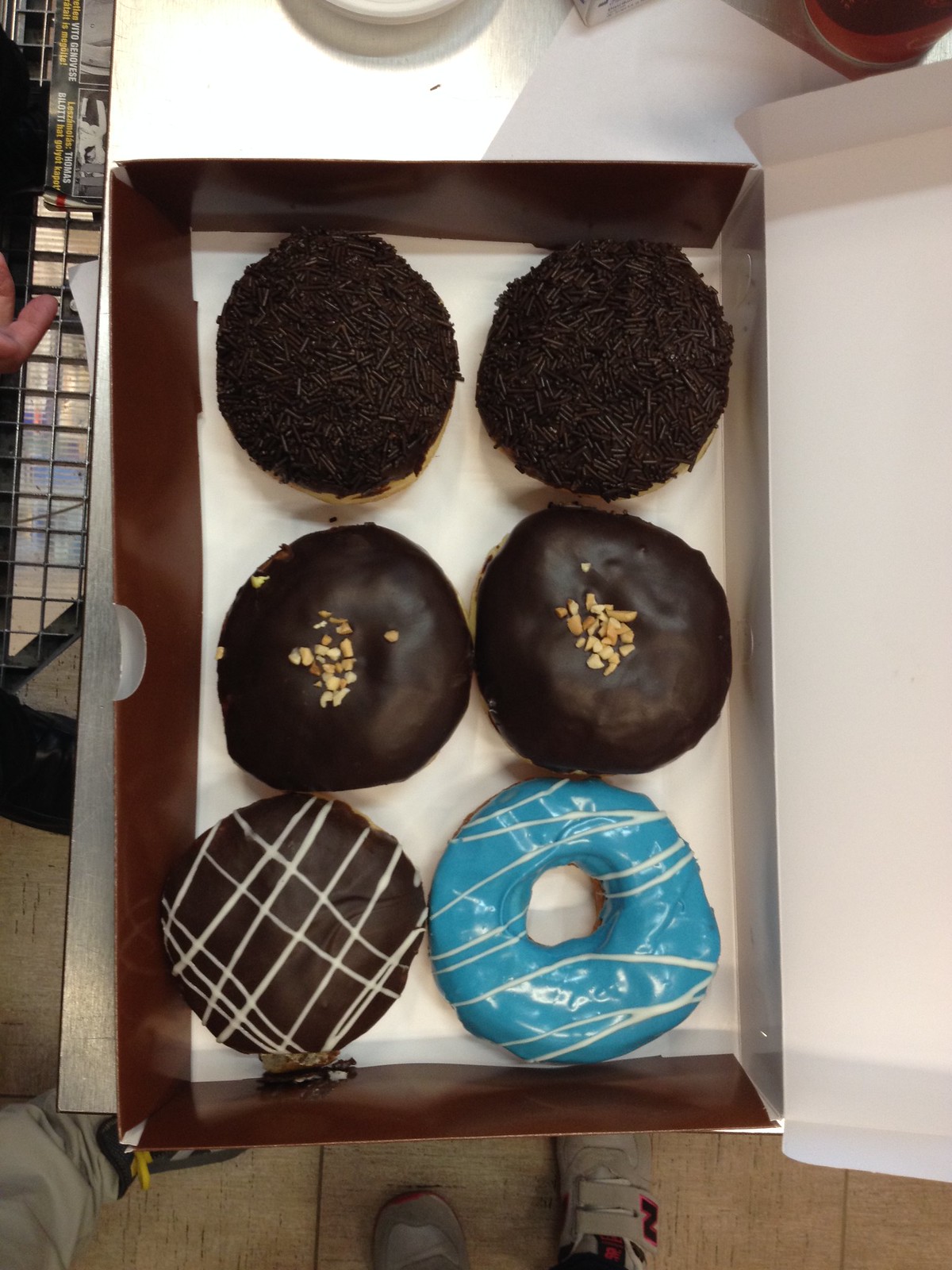This is a bird’s eye view photograph of six doughnuts in an open box, which is brown on the outside and white on the inside. The box is positioned longways and lies on a wooden table. Starting from the top are two dark brown doughnuts heavily covered in chocolate sprinkles. In the middle, there are two chocolate frosted doughnuts with no holes, instead adorned with peanut shavings. On the left side of the box is a chocolate doughnut with white icing stripes running across it, while on the bottom right is a blue doughnut also decorated with white icing stripes. The box is open, with its flap directed towards the right, and the scene is captured in portrait orientation. There are indistinct figures of people visible around the edges of the box, possibly observing the doughnuts.